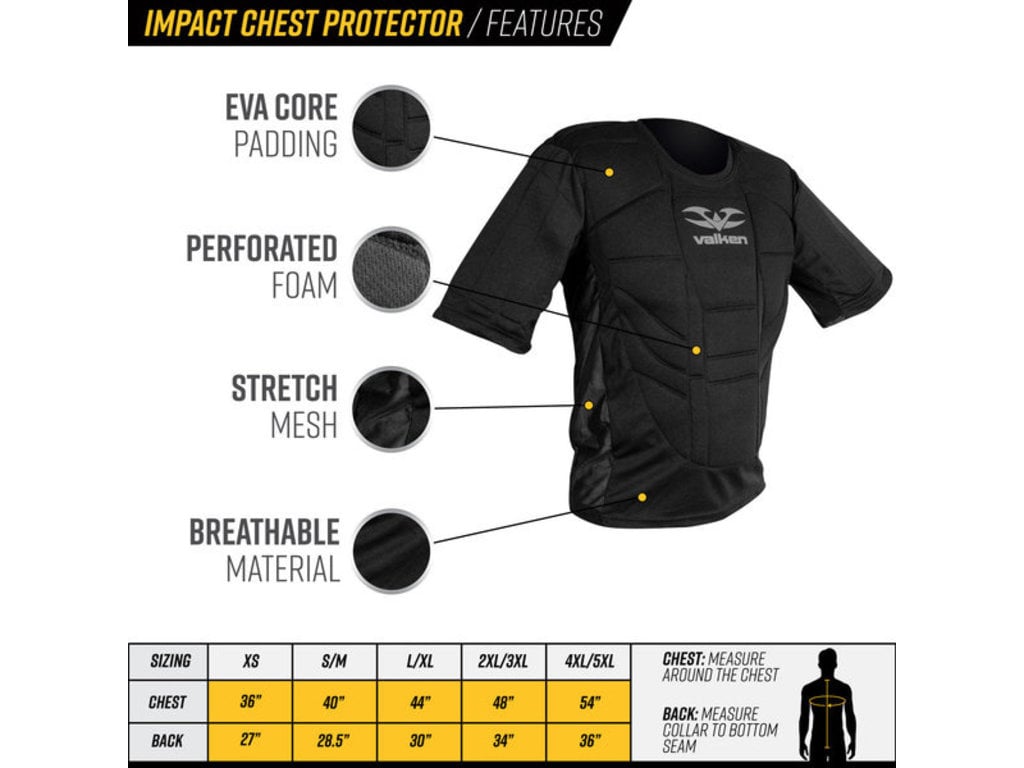The image showcases an "Impact Chest Protector" by Valken, prominently displayed against a black rectangle background. The text "Impact Chest Protector" stands out in yellow, while "Features" is written in white. The main visual features a padded, short-sleeve shirt designed for protection, embossed with the Valken brand logo in gray on the front. The image highlights key features: EVA core padding for impact protection, perforated foam near the stomach area for enhanced breathability, and stretch mesh on the sides for a customizable fit. Detailed close-ups of these materials branch out from the main shirt image. 

At the bottom, a comprehensive sizing chart offers a range from extra small (chest: 36 inches, back: 27 inches) up to 5XL (chest: 54 inches, back: 36 inches). Clear instructions are provided for measuring both chest circumference and back length, ensuring users can accurately determine their size for an optimal fit.